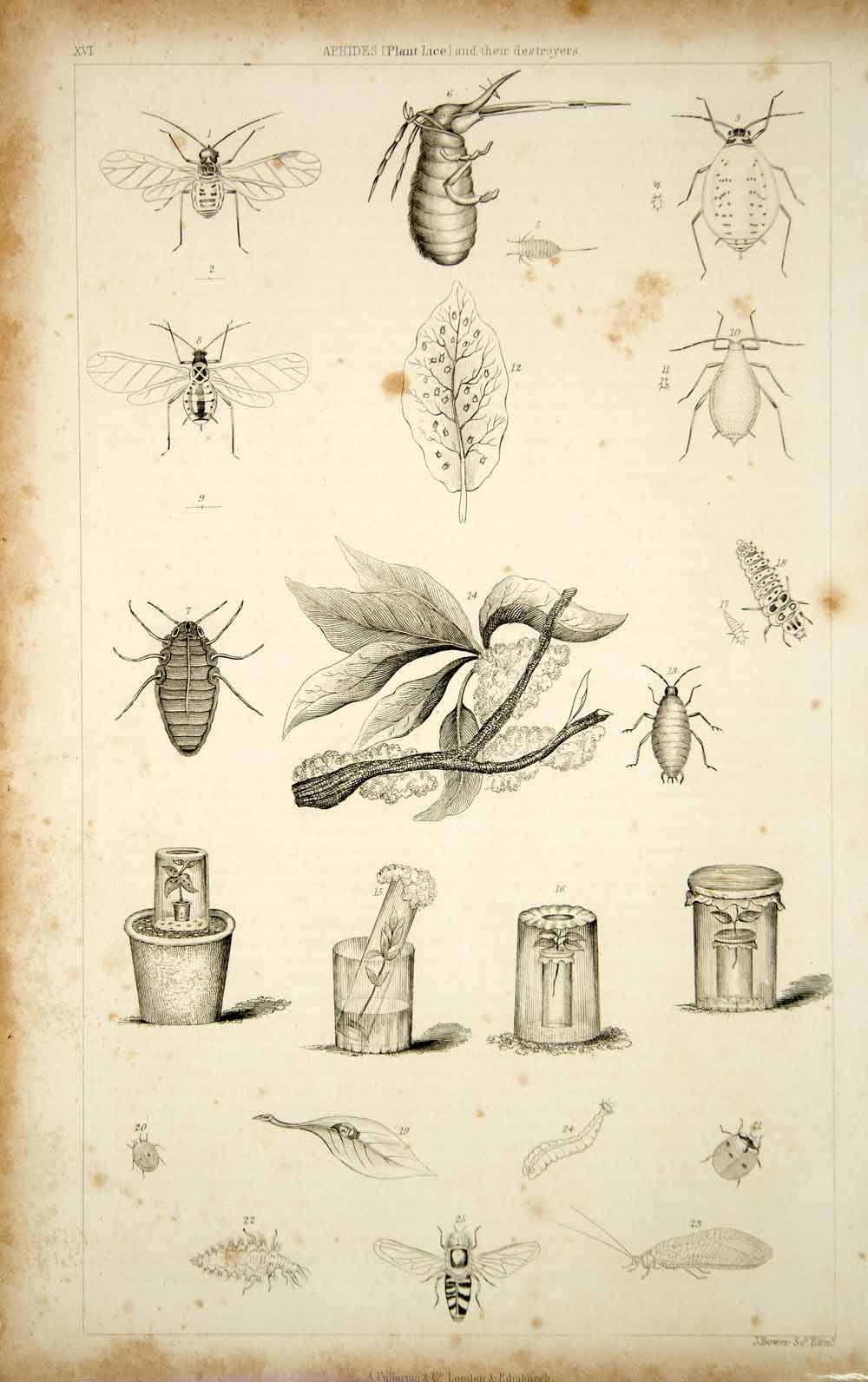The image features a page from an old, stained book that showcases a detailed ink illustration. At the top, the title reads "Aphides (Plant Lice) and Their Destroyers." The page is organized into rows brimming with intricate drawings of various bugs and plants. In the top-left corner, there's a fruit fly, followed by a beetle with a long spike, and what appears to be a ladybug in the top right. Below this, there's another bug resembling a fly. The middle of the page is dominated by a tree branch with leaves, and adjacent to it, a leaf infested with tiny bugs, as well as a chrysalis-like structure. 

As we move down, the next row presents three more insects, including some that look like a beetle and a bug with wings, along with additional leaves. The illustrations in the fourth row depict different methods to start growing a plant from a seed, shown through various containers and solutions—perhaps dips or coverings to combat the pests. In the final row, there are more bugs, a bee, a caterpillar-like creature, and another bug on a leaf. Altogether, these finely detailed line drawings offer a meticulous exploration of both pests and plants, reflective of the page’s antiquated nature and educational purpose.